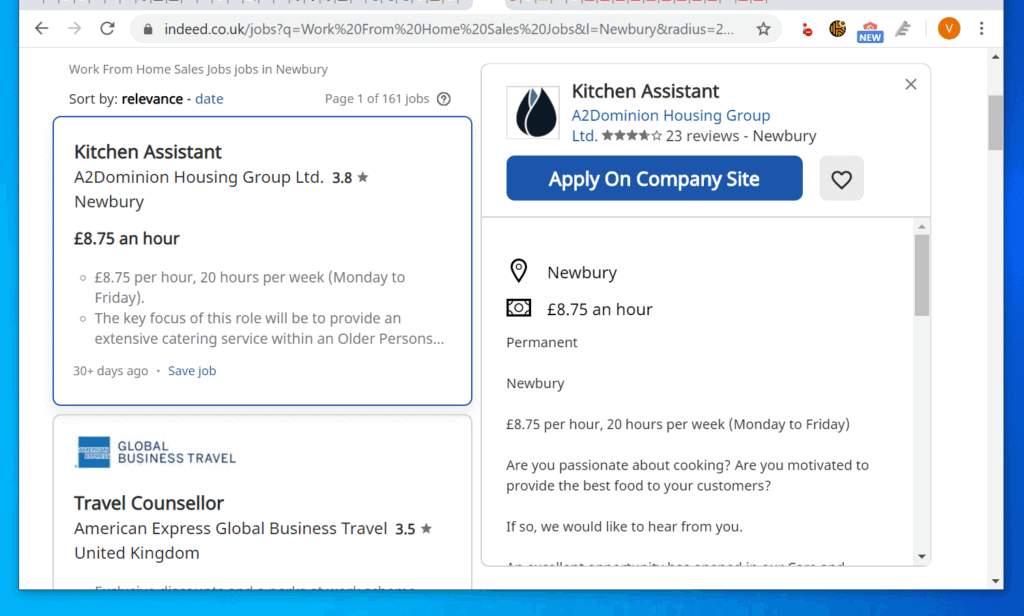The image showcases a job search page on the Indeed website (indeed.co.uk/jobs), specifically focused on "work from home sales jobs in Newbury." At the top of the page, there are navigation buttons including back, forward, and refresh arrows. 

The search results display the first page out of 161 possible pages, listing various job opportunities. The first job listing is for a "Kitchen Assistant" at A2 Dominion Housing Group Limited, rated 3.8 stars. This position is located in Newbury, offering a pay rate of £8.75 per hour for a 20-hour workweek, Monday to Friday. The role primarily involves providing extensive catering services for older persons. This listing was posted over 30 days ago.

The second listing is for a "Travel Counselor" at American Express Global Business Travel, rated 3.5 stars and based in the United Kingdom. However, part of the listing is cut off and incomplete.

On the right side of the screen, the Kitchen Assistant job details are prominently displayed with a large, blue "Apply on company site" button featuring white text. Below this, the job's compensation and work hours are reiterated: £8.75 per hour for 20 hours per week on a permanent basis.